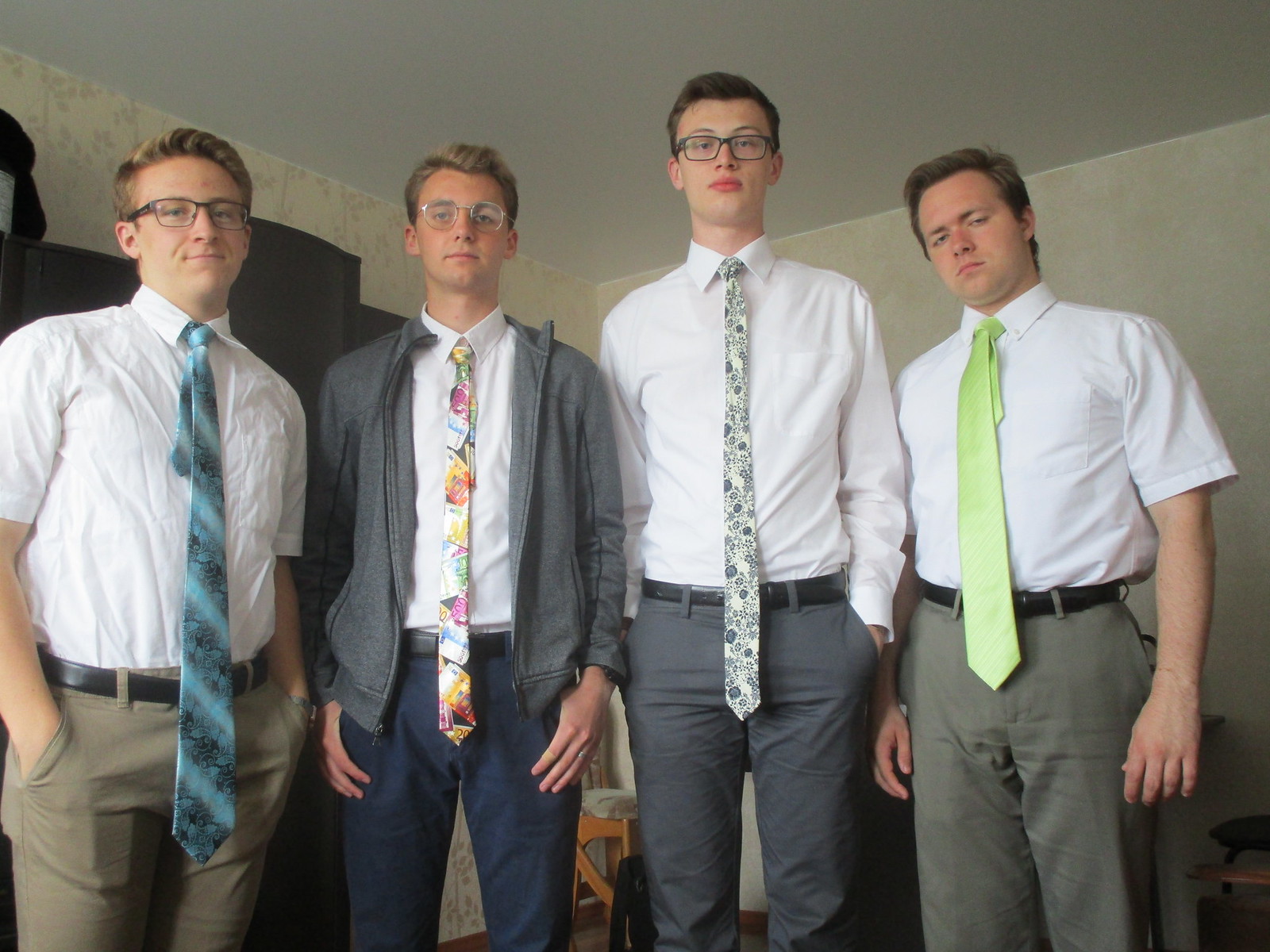In this photograph, four young men, likely teenagers or in their early 20s, are dressed in semi-formal attire and are standing in a minimalist white bedroom. Each man is wearing a white dress shirt paired with dress pants, and they all sport black belts. The two men on the outside are dressed in short-sleeved shirts, while the two in the middle wear long sleeves. 

On the far left, a man with blondish brown hair and brown-framed glasses wears khaki pants and a striking blue tie with black stripes that extends past his pubic area. Next to him, the man in a partially unzipped grey sweater and silver-framed glasses dons dark blue pants with a multicolored floral tie in shades of pink, blue, and orange, which also extends past his pubic area. 

Moving to the right, the third man, who has black-framed glasses, is dressed in grey pants and a tie featuring a black and white floral pattern stretching past his pubic area. Finally, the far-right man, distinguished by his lack of glasses, wears olive-colored pants and a vivid lime green tie that reaches just above his pubic area. 

All four have short haircuts that are above their ears, contributing to the professional, albeit quirky, look created by their ensemble of unusually long, colorful ties.